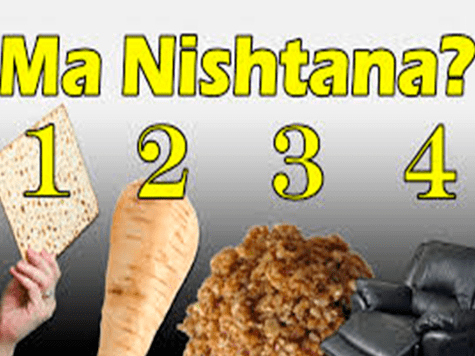The image features a PowerPoint slide with a gradient background transitioning from black at the bottom to white at the top. The slide includes four numbered objects arranged horizontally across the slide. 

1. On the far left, a hand is holding a large square piece of pita bread by the bottom corner, with a yellow number "1" superimposed on the top half of the bread.
2. To the right of the pita, there is a partial giant carrot, missing its tip, marked with the number "2."
3. Midway to the right, the number "3" designates an object resembling brown, bushy coral, which could be interpreted as having a fibrous, wool-like, or yarn-like texture.
4. On the far right, the number "4" is placed above a black recliner chair, resembling a barco lounger or lazy boy.

At the top of the slide, the text "Ma Nishtana?" is displayed, suggesting a question. The colors in the image include various shades of gray, black, yellow, tan, orange, and brown. The overall composition of the slide hints at a visual questionnaire or advertisement, possibly in a different language.